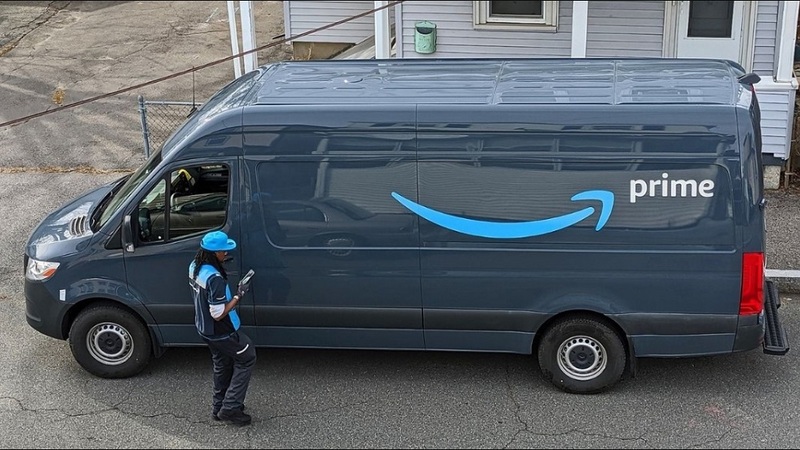A man is standing next to the passenger door of a glossy Amazon Prime delivery van, which is prominently featuring the iconic Amazon smile and "Prime" in white letters. He is wearing a bright blue baseball cap that matches the Amazon smile logo and a distinctive short-sleeved shirt. The shirt has a complex color scheme: bright blue on the back, upper shoulder area, and down the center of the chest; dark blue on the sides; and medium gray-blue on the back and arms. The colors of the van and the shirt blend harmoniously, especially the gray on the arms that mirrors the van’s hue. The man is holding a smartphone or possibly a tracking device used for deliveries, such as mapping, routing, or check-ins. The van is a larger, taller model, parked facing to the right. Behind it, a small wooden house with a chain-link fence is visible. The photograph seems to have been taken from the second or third floor of a building across the street. The image captures a daytime scene with some shadowing, suggesting it’s a semi-cloudy day.